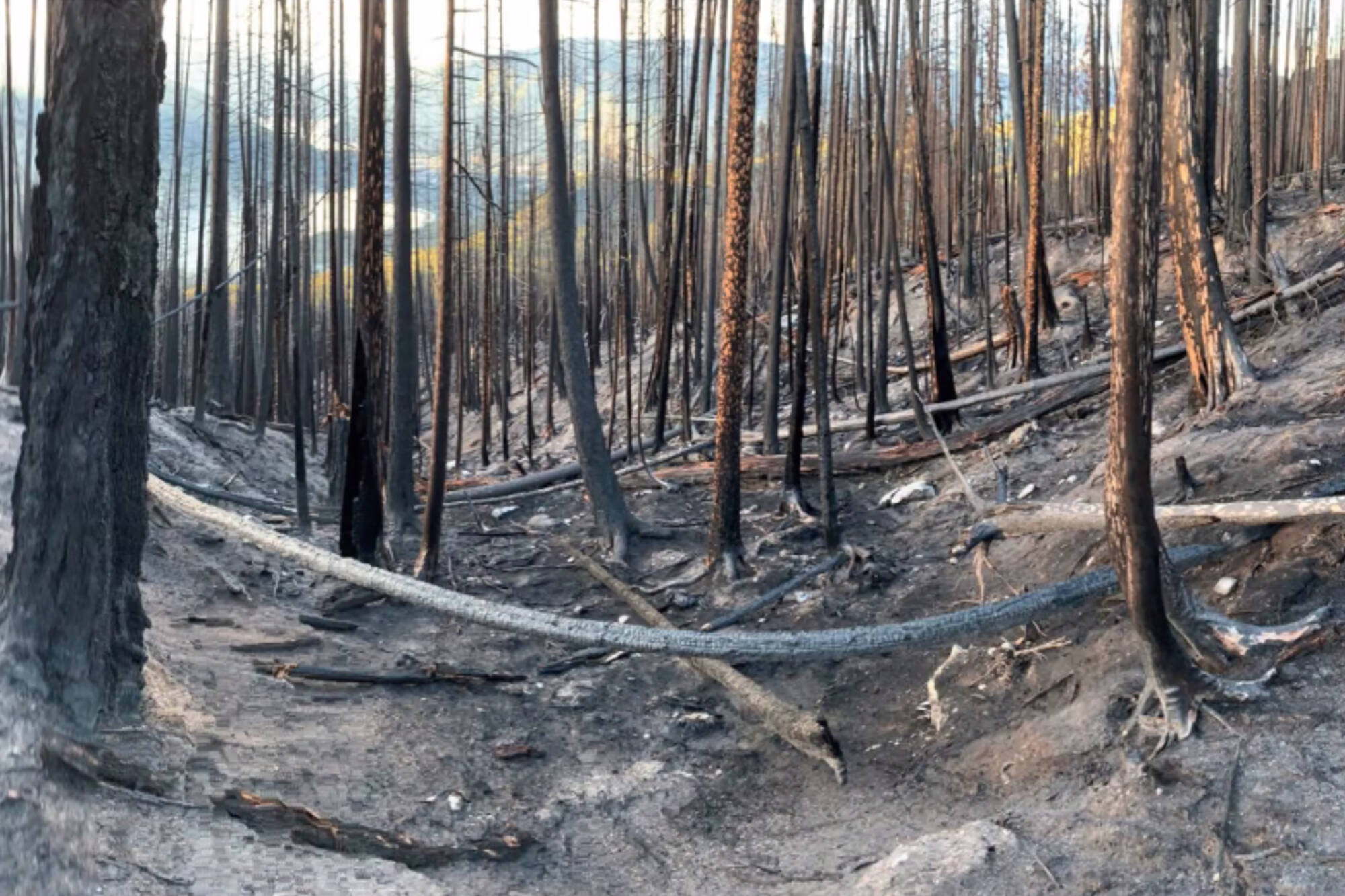The image depicts a desolate forest landscape, starkly characterized by numerous thin, barren trees. The scene is somber, with the trees appearing either burned or stripped of their limbs, contributing to an overall sense of devastation. The forest floor is void of grass or underbrush, instead covered in ash, dirt, and mud, indicating the aftermath of a forest fire. Among the charred landscape, several tree stumps and fallen trees are visible, further emphasizing the destruction.

In the background, partially obscured by the dense array of trees, lies a mountainous hillside. The hill continues the pattern of burned trees, extending the devastation across the terrain. Interestingly, in the distant background, you can make out a contrasting scene where lively green trees and possibly a lake suggest untouched areas not reached by the fire. The sky above is filled with dreary gray and blue clouds, tinged with the colors of a setting sun, adding to the bleak yet serene ambiance. The scene is devoid of any wildlife or human presence, reinforcing the solitude and desolation of this deep forest environment.